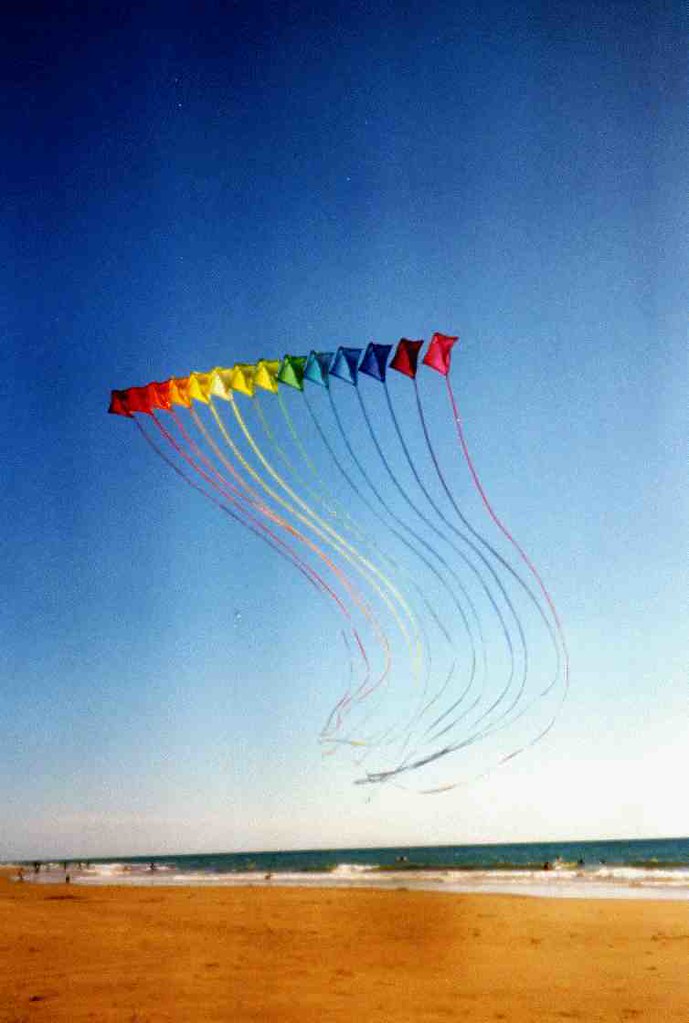The image captures a serene beach scene with orange-hued sandy shores occupying the bottom quarter of the frame. Just above the shore, a sliver of a calm, teal-green ocean meets the sand, its waves gently crashing and displaying frothy white crests. The top three-quarters of the photo reveal a vast blue sky with a slight haze and a few scattered clouds.

Dominating the middle of the image, an array of 13 kites forms a vivid rainbow gradient that transitions smoothly from dark red on the left to pink on the right. These kites, each diamond-shaped with very long, flowing tails that curl and move in an S-shape, are striking against the clear sky. The colors of the kites and their tails create a spectacle, moving through shades of red, orange, yellow, green, blue, indigo, and violet.

In the distance to the left, a few indistinct figures can be seen on the beach, adding a subtle touch of human presence to the tranquil scene. The overall image, despite a slight grainy quality, beautifully showcases the colorful kites and the peaceful beach environment.